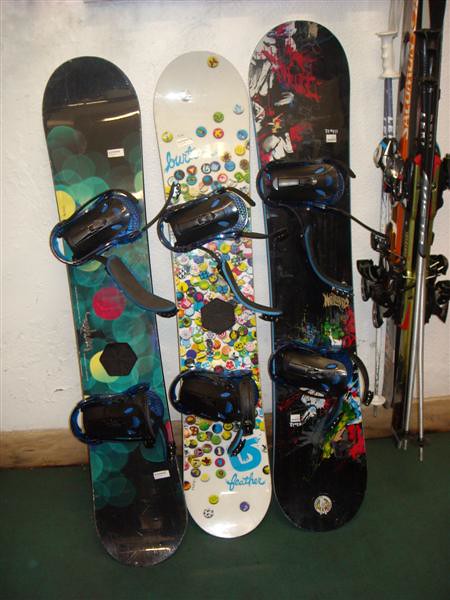The photo features three vibrant snowboards standing upright against a plain white wall with a wooden baseboard. The floor beneath them is painted a striking green. To the right of the snowboards, ski poles—likely for snowboarding or skiing—are also leaning against the wall.

Each snowboard is equipped with footholds, which are black with blue accents. The snowboard on the left is predominantly black, adorned with a variety of geometric shapes, including light green, bright red, and yellow circles. These shapes are dotted across the board, creating a dynamic pattern focused mainly in the center. The middle snowboard stands out with its white base, decorated with numerous small, vividly colored circles that cluster towards the center and disperse towards the edges. At the bottom, a blue logo features white lettering and cursive writing. The snowboard on the right is primarily black, featuring a vibrant, irregular design of paint splatters in shades of red, green, blue, white, and yellow, giving it a graffiti-like appearance.

This colorful array of snowboards is complemented by ski poles neatly positioned nearby, adding to the overall impression of a well-organized snow sporting setup.